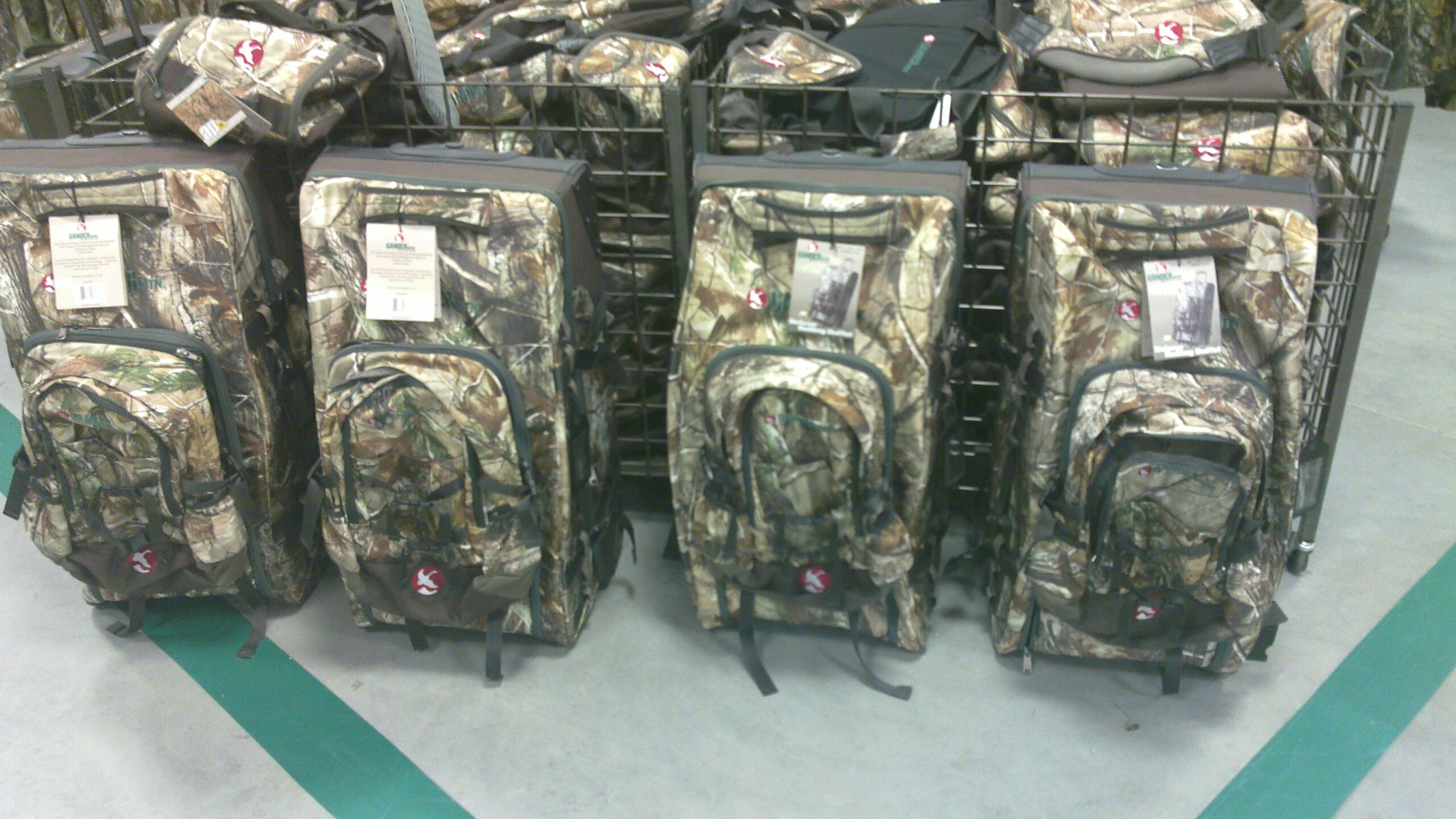In this indoor store setting, a collection of camouflage-themed hiking or hunting backpacks is prominently displayed. The floor beneath them is made of white tiles adorned with teal and green stripes. At the forefront, four backpacks stand upright, showcasing their intricate nature-inspired camouflage patterns, which include branches, sticks, grass, and leaves, designed to blend seamlessly with woodland environments. Each backpack bears a red circle emblem featuring a white bird and is tagged with a manufacturer's label that includes pricing and barcodes. Behind these, a sturdy brown metal crate is filled with many more of these camouflage backpacks, stacked neatly within. The overall scene captures a detailed display of large, nature-themed backpacks, ideal for outdoor activities like hunting or hiking.